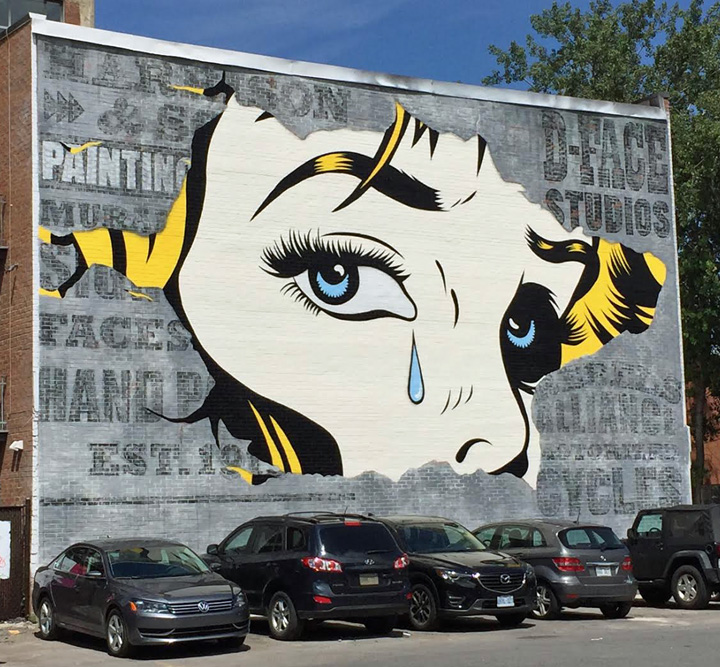The image captures a striking mural on the gray side of a building. This vibrant piece of art features an animated, comic book-style close-up of a woman's face, focusing mainly on her eyes, nose, eyebrows, and right cheekbone. The woman has striking blue eyes with a single blue tear streaming down from her right eye, long eyelashes, and blonde streaks in her hair. Her skin is depicted in a porcelain white hue. The mural appears almost three-dimensional, as if the woman's face is emerging from the wall. Painted or printed on the backdrop are the words "D Face Studios" in the upper right corner. In front of this mural, there are five parked cars. The first is a sedan, followed by two SUVs, a hybrid car, and a black Jeep, forming a typical city parking lot scene. The overall composition blends the vibrant artistry of the mural with the everyday reality of urban life.